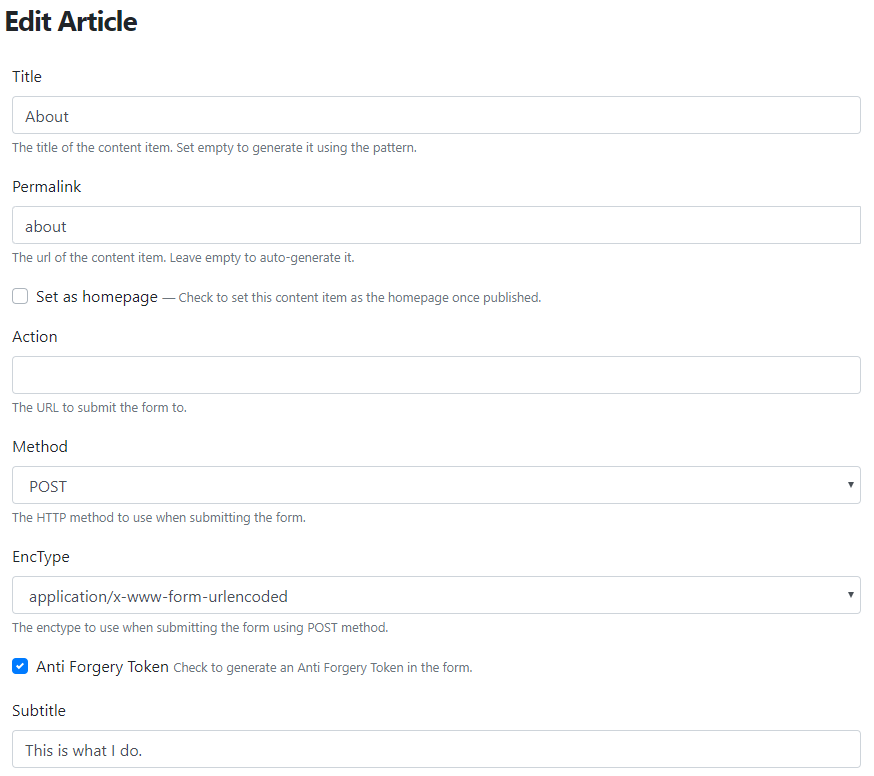The screenshot features a white background with black text that outlines the layout of a form editing interface. At the top of the form, the text "Edit Article" is displayed. Below this, there are fields labeled "Title" and "About," guiding the user to input the title of the content item and an optional description, with a note that leaving the title field empty will auto-generate a title based on a set pattern.

Further down, a "Permalink" field is provided, accompanied by guidance to leave it empty if an auto-generated URL is preferred. An unchecked checkbox labeled "Set as homepage" is present, which, when selected, would set the content item as the homepage upon publication.

The form continues with sections for the form submission URL ("Action") and the HTTP method to use ("Method"), which is set to "Post." There is a drop-down arrow next to the method selection. Additionally, another drop-down menu is available for selecting the "ENC type," which is set to "application/x-www-form-urlencoded."

A checked checkbox titled "Anti-forgery token" indicates that an anti-forgery token will be generated for the form. The final field visible is labeled "Subtitle" with the entry "This is what I do."

Absent from the image are any photographic or illustrative elements, and there are no depictions of people, animals, birds, plants, flowers, trees, or automobiles.